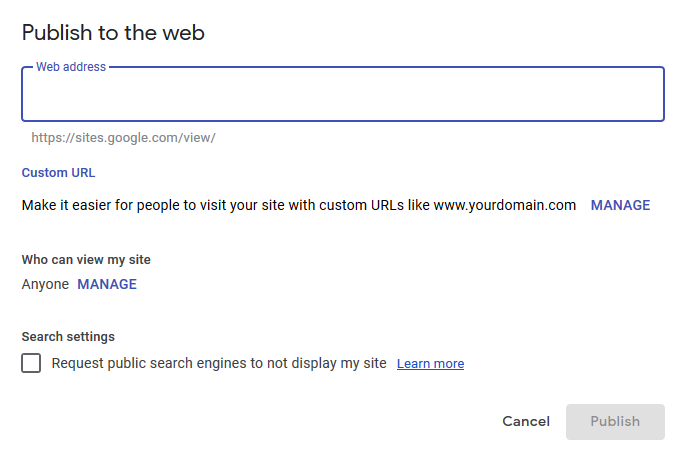This image depicts a Google Sites interface for publishing a site to the web. Central to the image is a long input box labeled "Web address," where users are prompted to enter a URL. Below this field, there's the typical format for a Google Sites address: "https://sites.google.com/view/". Adjacent to this area, there is a section labeled "Custom URL," explaining how users can create more accessible web addresses like "www.yourdomain.com." This section includes the word "Manage" in blue, indicating an actionable link.

Further down, another section titled "Who can view my site" displays the option "Anyone," alongside a blue "Manage" link, allowing the user to adjust visibility settings. Additionally, there's an area marked "Search settings," which features a checkbox option for "Request public search engines to not display my site." Next to this option is a "Learn more" link in blue with an underline, suggesting further information is available.

The entire interface is presented on a clean, white background with essential information highlighted in black print. Key interactive elements like "Manage" and "Learn more" are in blue text to attract attention. Overall, the design is straightforward and functional, emphasizing user-friendly navigation with clear calls to action.